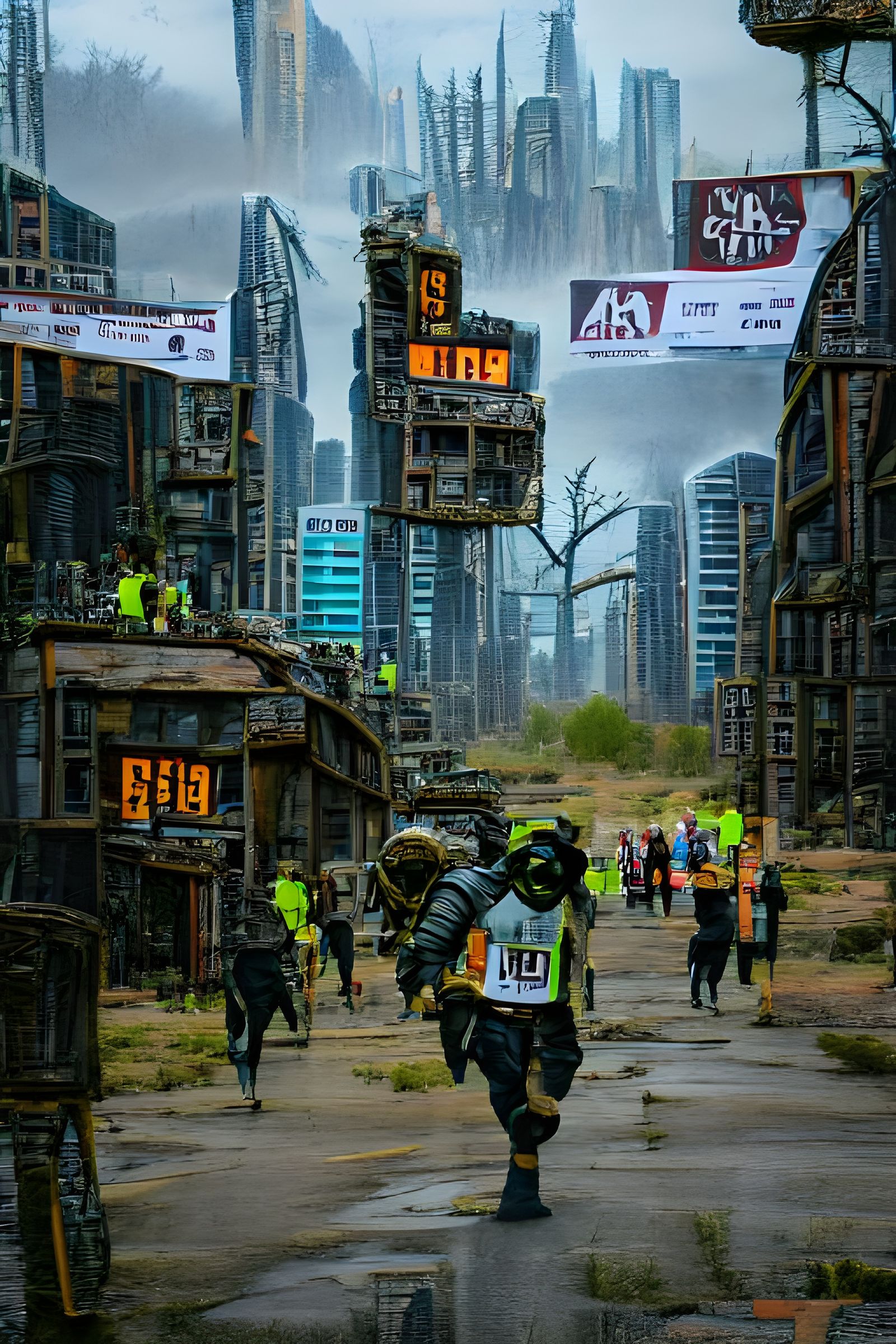The image is a detailed painting depicting a dystopian city scene. In the background, a foggy and smog-filled sky looms over a tall skyline of silver, metallic, and dark-colored high-rise buildings. The foreground features a street in disarray, with weeds and tall grasses growing from cracks in the pavement. People clad in bright green and orange protective gear are scattered throughout the scene, running amidst the chaos. Some of these figures, which appear to be slightly exaggerated and possibly non-human, are also seen on the rooftops of nearby buildings. Signage in the background includes white signs with red markings, though the text is illegible. Overall, the chaotic scene conveys a sense of frantic activity and urban ruin.